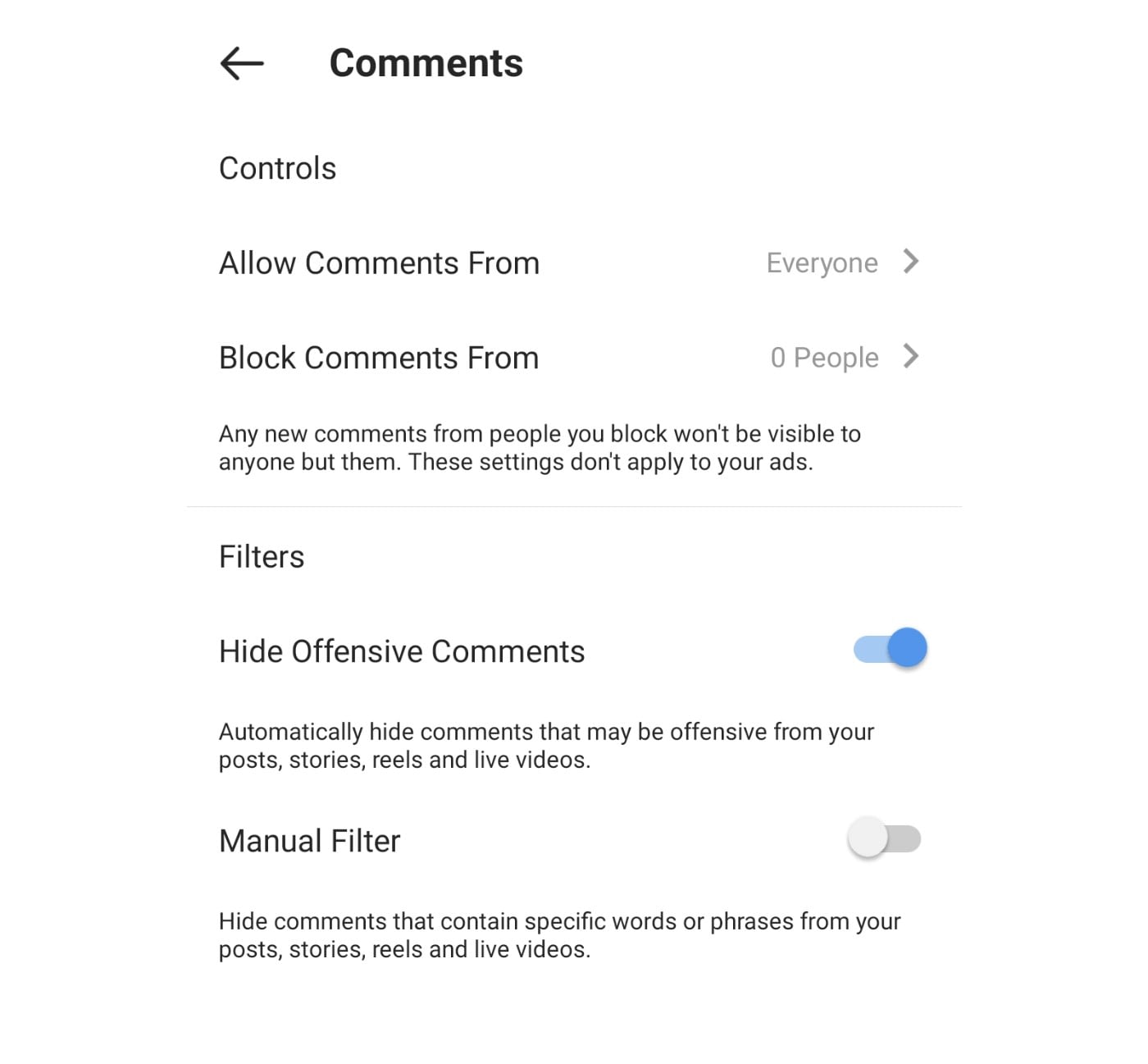This is a detailed screenshot of a website's comment control settings page. At the top of the page, there is a navigation option indicated by a black left-pointing arrow next to the word "Content," which is bold and in black letters. Below this is the heading "Controls."

Under "Controls," there is a section titled "Allow comments from," with a dropdown menu beside it showing the option "Everyone" in grey letters accompanied by a right-pointing arrow. Directly below this is the section "Block comments from," displayed in black letters, with a dropdown menu next to it that reads "0 people" in grey, also with a right-pointing arrow.

Following this is a small paragraph in black letters that reads: "Any new comments from people you block won't be visible to anyone but them. These settings don't apply to cats." This is separated from the next section by a faint grey line.

The next section is labeled "Filters." Within this section, there is the option to "Hide offensive comments," with a toggle button next to it that is turned on and appears blue. This setting description reads, "Automatically hide comments that may be offensive from your posts, stories, and live videos."

Below this is the "Manual filter" option in black letters, alongside a toggle button that is not turned on. The description for this option reads: "Hide comments that contain specific words or phrases from your posts, stories, reels, and live videos."